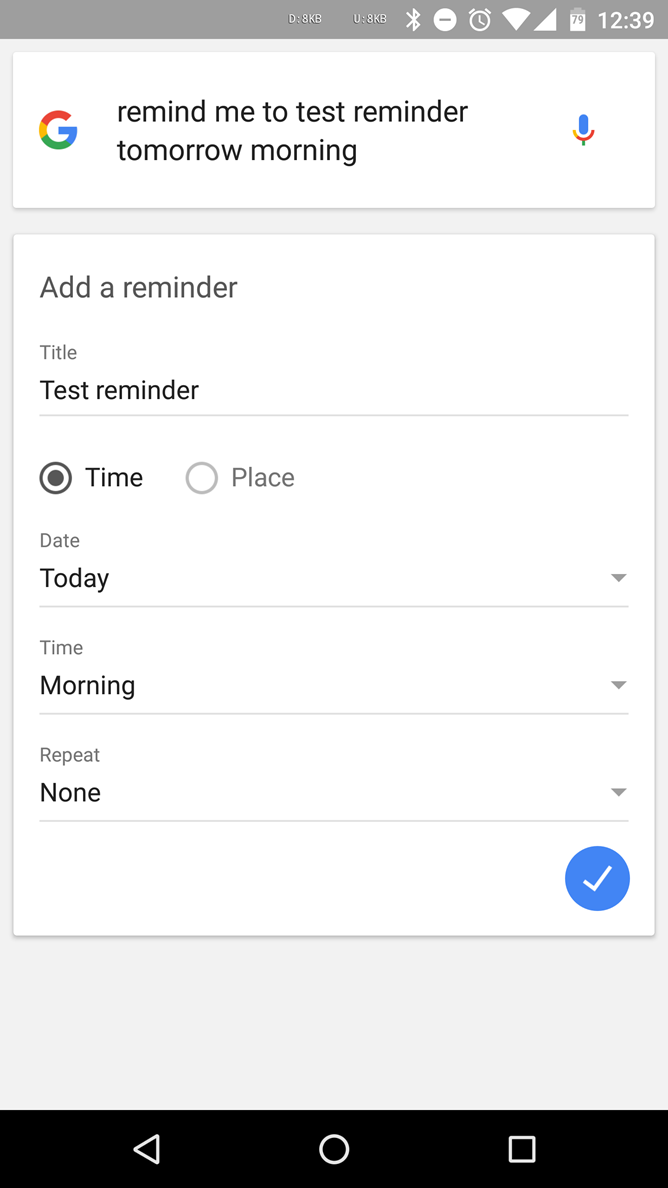This is a detailed description of a screenshot taken from a phone. At the top of the screen, there is a grey status bar displaying various icons. In the center of this bar, "D: 8KB" and "U: 8KB" are shown, which likely indicate data usage statistics. To the left, there are icons for Bluetooth and Do Not Disturb (the latter being active). On the right side of the status bar, there are icons for cellular signal (fully filled), Wi-Fi (fully filled), and battery level (at 79%). The time "12:39" is also displayed on the far right.

Below the status bar, a rectangular banner contains the Google logo, presented in its familiar red, blue, green, and yellow colors, followed by a text command: "Remind me to test reminder tomorrow morning." At the very right of this banner, there is a microphone icon.

Underneath the banner, the interface prompts the user to "Add a reminder." The placeholder text "Title" is visible, and below it, the text "Test reminder" is entered, separated by a line.

Further down, sections for setting the reminder include "Time" and "Place." The "Time" option is selected, indicated by a black dot within a circled area, though the circle is not fully filled. The "Place" option next to it shows an empty circle.

Further down the interface, the user can select the reminder's "Date" with "Today" as the default option, accompanied by a drop-down arrow on the right. Another line separates this section from the "Time" section, preset to "Morning." Similarly, the "Repeat" section is set to "None," with drop-down arrows accompanying both options.

At the bottom right of the screen, there is a blue circle with a white check mark inside.